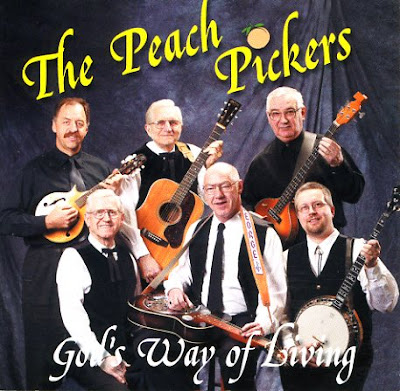This is an album cover of a band called The Peach Pickers. The title "The Peach Pickers" is displayed at the very top in yellow writing, with a peach symbol cleverly used as the dot over the "i." The album's name, "God's Way of Living," is written at the bottom in white. The image features six older gentlemen, all holding different stringed instruments such as an acoustic guitar, mandolin, banjo, bass guitar, and steel lap guitar. They are dressed primarily in black and white attire and are positioned in front of a grey studio backdrop, looking and smiling towards the camera. The gentleman on the left wears a black long-sleeve shirt and plays the bass guitar, the top middle gentleman dons a black vest and white long-sleeve shirt while holding an acoustic guitar, and the man to the top left, dressed in a black shirt and tie, holds a mandolin. The middle character, also in a black vest and white shirt with a black tie, holds the lap steel guitar. The overall setting is a posed studio photograph with square dimensions, accentuating the timeless and classic style of the cover.